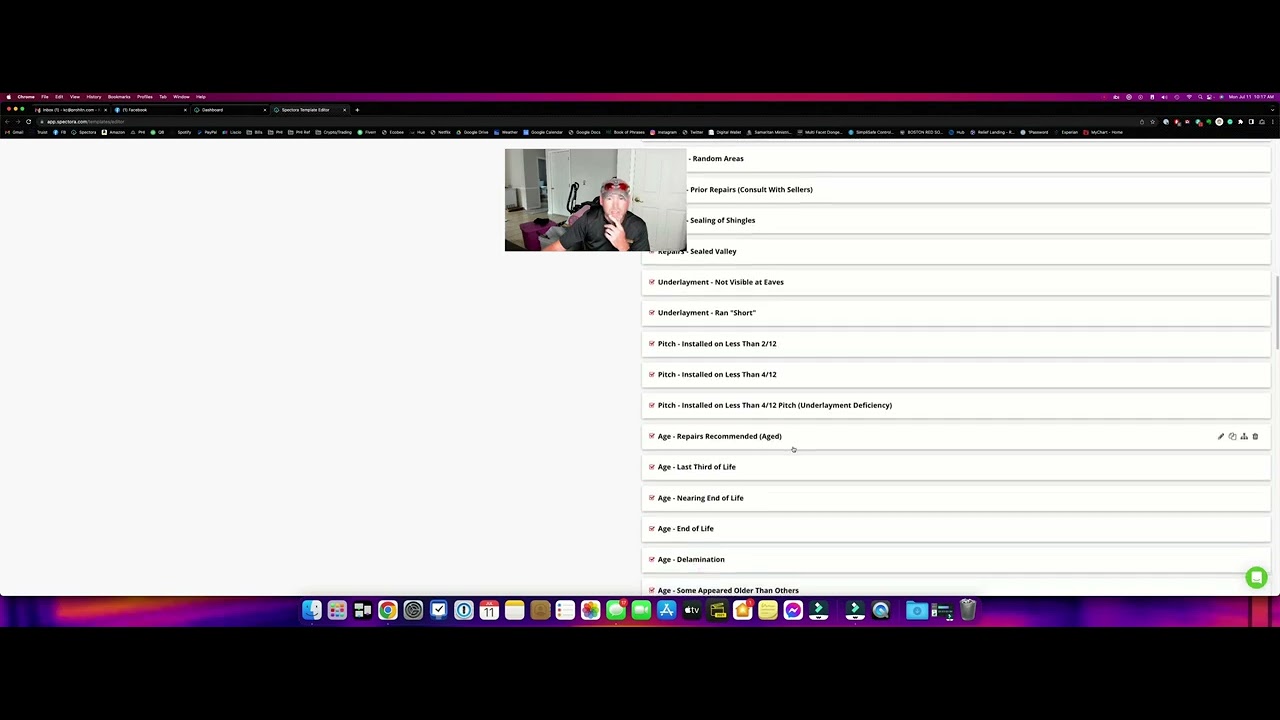The image displays a complex digital interface with numerous smaller elements that are difficult to decipher due to their size. The top of the screen features a black header with a long purple line running horizontally. This line appears to lighten towards the center. Along the left and right edges of this header, there are tiny white words that remain illegible despite enlargement attempts. 

Below the prominent header, three colored dots—red, yellow, and green—are visible, resembling typical window control buttons found in many applications. A search bar, filled with dark gray text in white font, is located below these dots. It appears there are five such search bars in total. To the far right of the screen, a series of tiny icons can be seen, though they are too small to identify specifically.

A portion of the lower section of the screen contains more black background with unreadable white text. Below this section, a larger image of a man wearing a baseball cap is shown. He appears to be in a room with grey walls and shiny, blonde-wood floors. The caption beneath this image reads: "Random areas prior repairs consult with sellers."

Below this visual, two white banners display more detailed text about inspection notes and recommendations, particularly concerning roof conditions and repairs. These notes include terms such as "shingles repairs," "sealed valley," "underlayment not visible at eaves," and various mentions of "pitch," such as "installed on less than 212 pitch" and "underlayment deficiency." Keywords like "age repairs recommended," "aged," "last third of life," "nearing end of life," and "end of life" indicate the state and recommended interventions for the roof's materials. Each note is accompanied by a small purple box with a checkmark.

Towards the bottom left of the image, flashes of orange and purple are interspersed with several small app icons. These icons include Google Chrome, a calendar marking January 11th, a note-taking app, Google Chat, and Google Photos, spread across a black lower section of the interface.